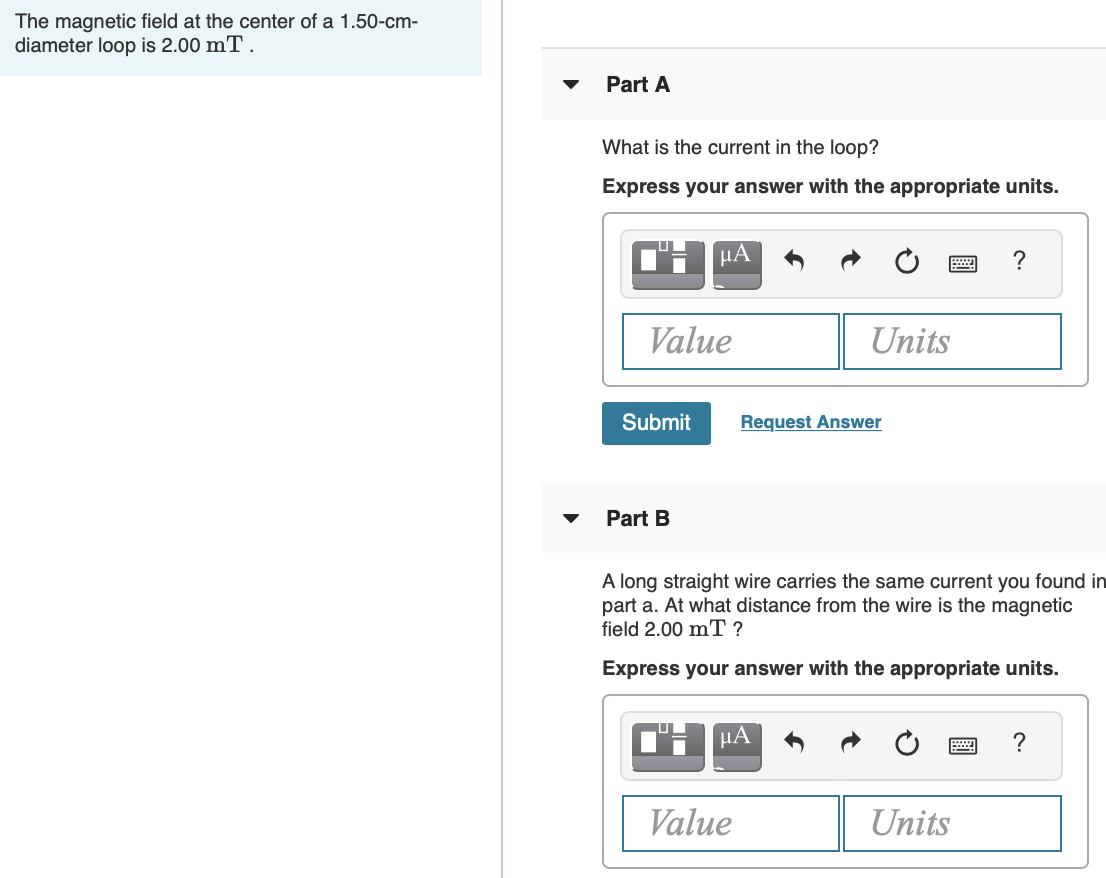The image is sectioned into two distinct parts. On the first side, a small bluish-gray box contains black text stating, "The magnetic field at the center of a 1.50 centimeter diameter loop is 2.0 mT." This text is positioned toward the top of the section. A gray vertical line divides the image centrally. 

In the first section below the text box, a gray banner with black text reads "Part A," followed by a dropdown menu. Black text prompts the user with the question, "What is the current in the loop?" Underneath, bold black text instructs to "Express your answer with the appropriate units." Beneath this, there are seven clickable symbols arranged horizontally. Below these symbols, there is a box for entering the numerical value of the answer and another box for entering the units. At the bottom of this section, there is a blue button labeled "Submit" in white text and an underlined hyperlink that reads "Request Answer."

The second section mirrors the layout of the first. It features another gray banner with black text stating "Part B," accompanied by a dropdown menu. The prompt here asks, "A long straight wire carries the same current you found in Part A. At what distance from the wire is the magnetic field 2.0 mT?" It similarly instructs to "Express your answer with the appropriate units." As in Part A, this section includes seven clickable symbols, a value input box, and a units input box.

Overall, the layout is structured to guide users through understanding the magnetic field properties and calculating the necessary current and distance metrics with clear, step-by-step prompts.